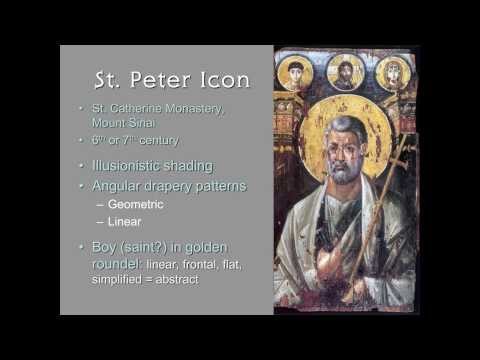The image is a PowerPoint presentation slide with a black background, featuring an ancient painting of Saint Peter on the right side. The painting, which appears to be from a church, depicts Saint Peter with a yellow halo around his head, holding a crook. Above his head, there are three small circles with faces of other saints or venerated figures. On the left side of the slide is text with the title "Saint Peter Icon" and a bulleted list that includes: "Saint Catherine Monastery, Mount Sinai", "6th or 7th Century", "Illusionistic Shading", "Angular Drapery Patterns", and sub-points "Geometric and Linear". Another bullet point states "Boy (Saint?) in Golden Roundel: Linear, Frontal, Flat, Simplified = Abstract". The painting is described to be around four inches wide by three and a half inches tall, set on a black bordered background.